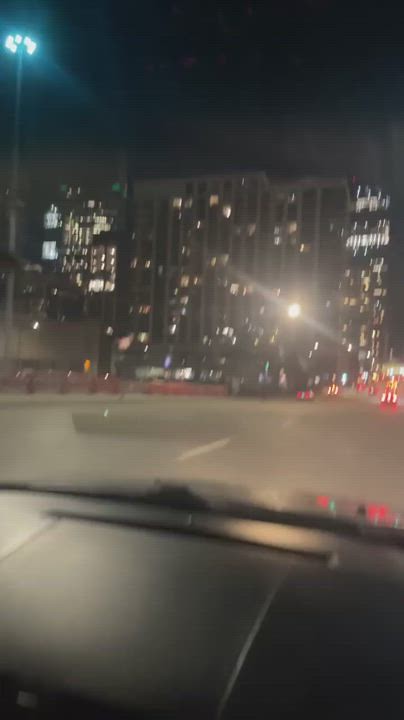A blurry nighttime photograph taken from inside a vehicle showcases a black dashboard and a view through the windshield. The scene outside reveals a bustling city environment with a large office building displaying a mix of illuminated and darkened windows. Central to the photograph, a bright streetlight casts a bluish-white glow towards the buildings. The road ahead is adorned with orange construction barriers on the left and scattered traffic cones on the right, with one barrel conspicuously toppled over in the middle of the street. The sky outside is pitch black, accentuating the array of lights from surrounding vehicles and infrastructure. Multiple cars, their brake lights aglow, drive on the highway, contributing to the urban nighttime ambiance. The location is punctuated by the presence of distinct buildings that might include an office structure and a possible convention center. The overall scene evokes a lively yet constrained city atmosphere, perhaps reminiscent of Pittsburgh.